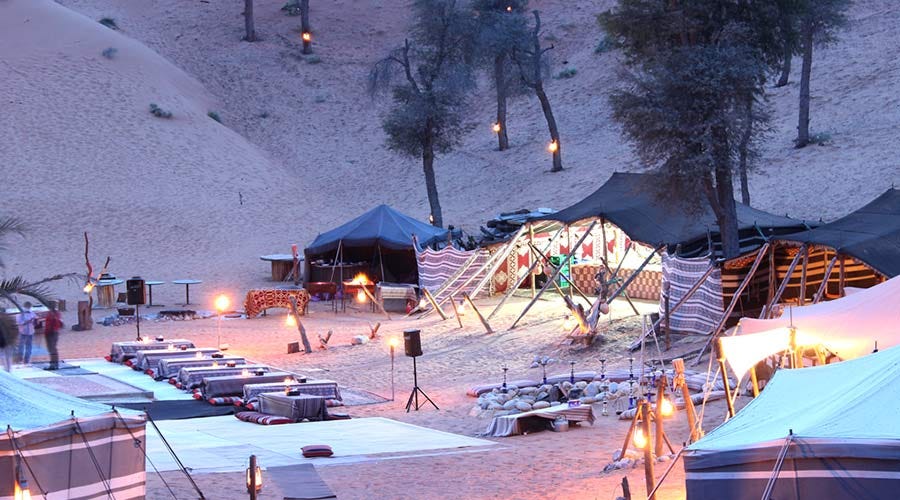The image depicts a rural outdoor scene covered in snow, interspersed with patches of sand. Tall trees, adorned with green leaves and hanging lanterns, surround the area, juxtaposing the stark wintry ground with their verdant foliage. Set in the middle of this picturesque setting is a small encampment, evocative of a tribal or historical recreation site. Seven tables, draped in cloths, are meticulously arranged—a block of six positioned linearly from left to right, with one set perpendicular at a 90-degree angle. The tables feature small, candle-based lamps, emanating a warm, inviting glow. Tents are pitched on the right side of the scene, with the soft luminescence of light visible from within two specific tents. In front of the tents, you notice benches or additional tables enhancing the communal feel of the space. Near the left edge, two individuals dressed in modern attire stand, adding a contemporary touch to this otherwise rustic, evocative tableau.